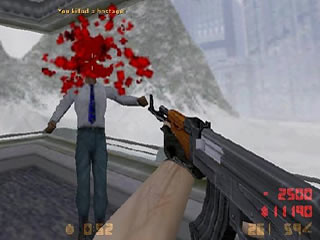The image depicts a graphic and violent scene, likely from a video game. In the lower left corner, a gun is prominently featured, marked with red numbers "2500" and "11190" beneath it. Another number, "2659," appears in a cream color. An arm holding an automatic rifle can be seen. In the foreground, a man dressed in black trousers and a white shirt with a blue tie is the apparent target. The man's head area is obscured by red splatters, implying a gunshot injury. The background shows a room bordered in white and possibly features grey mountains. The overall scene is quite disturbing and intense, indicating a high level of graphic violence typical in some video games.